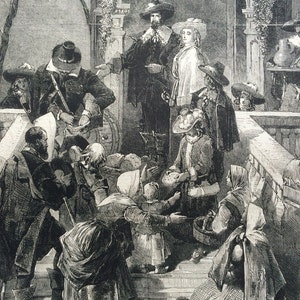In this black and white photograph, a dynamic and dramatic scene unfolds on an ornate, concrete staircase. The image, likely set in the 1600s or 1700s based on the attire, features a group of people including men, women, and children. The stairs are flanked by intricately designed columns and banisters reminiscent of castle architecture. Some of the individuals appear to be dressed as pirates; a man resembling Captain Hook, in a black hat and jacket, stands prominently near the top with a girl by his side, while another man on the left seems to be kicking someone down the stairs.

At different levels of the staircase, people are either standing, engaged in struggle, or falling. The varied expressions and actions add a chaotic energy to the scene. In the front of the image, a small child dressed in a cape stands out. Another noticeable figure is a woman in the front carrying a basket. The eclectic mix of ages and the disparity between those standing calmly and those in distress create a stark contrast, further enhanced by the absence of color in this historical photograph.